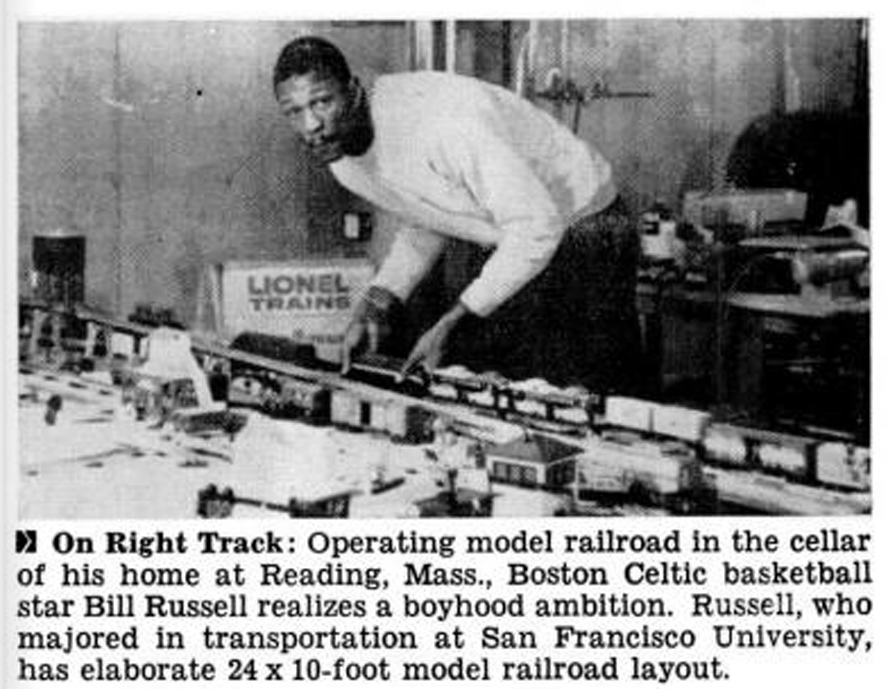This black and white photograph, originally appearing in a newspaper or article, captures Boston Celtic basketball star Bill Russell fulfilling a boyhood ambition by operating a model railroad in the cellar of his home in Reading, Massachusetts. Russell is seen leaning over an elaborate 24 by 10-foot model railroad layout, with train tracks running from left to right and a detailed diorama that includes tiny buildings and a water tower. He is wearing a long-sleeve white sweater and dark pants, and is holding a model train engine about the size of his hand. His dark hair is visible as he looks toward the camera. Behind him, a box labeled "Lionel Trains" can be seen, alongside a table with various objects on it against a gray wall. The caption below the image in black text reads: "On right track: Operating model railroad in the cellar of his home at Reading, Massachusetts, Boston Celtic basketball star Bill Russell realizes a boyhood ambition. Russell, who majored in transportation at San Francisco University, has an elaborate 24 by 10 foot model railroad layout."